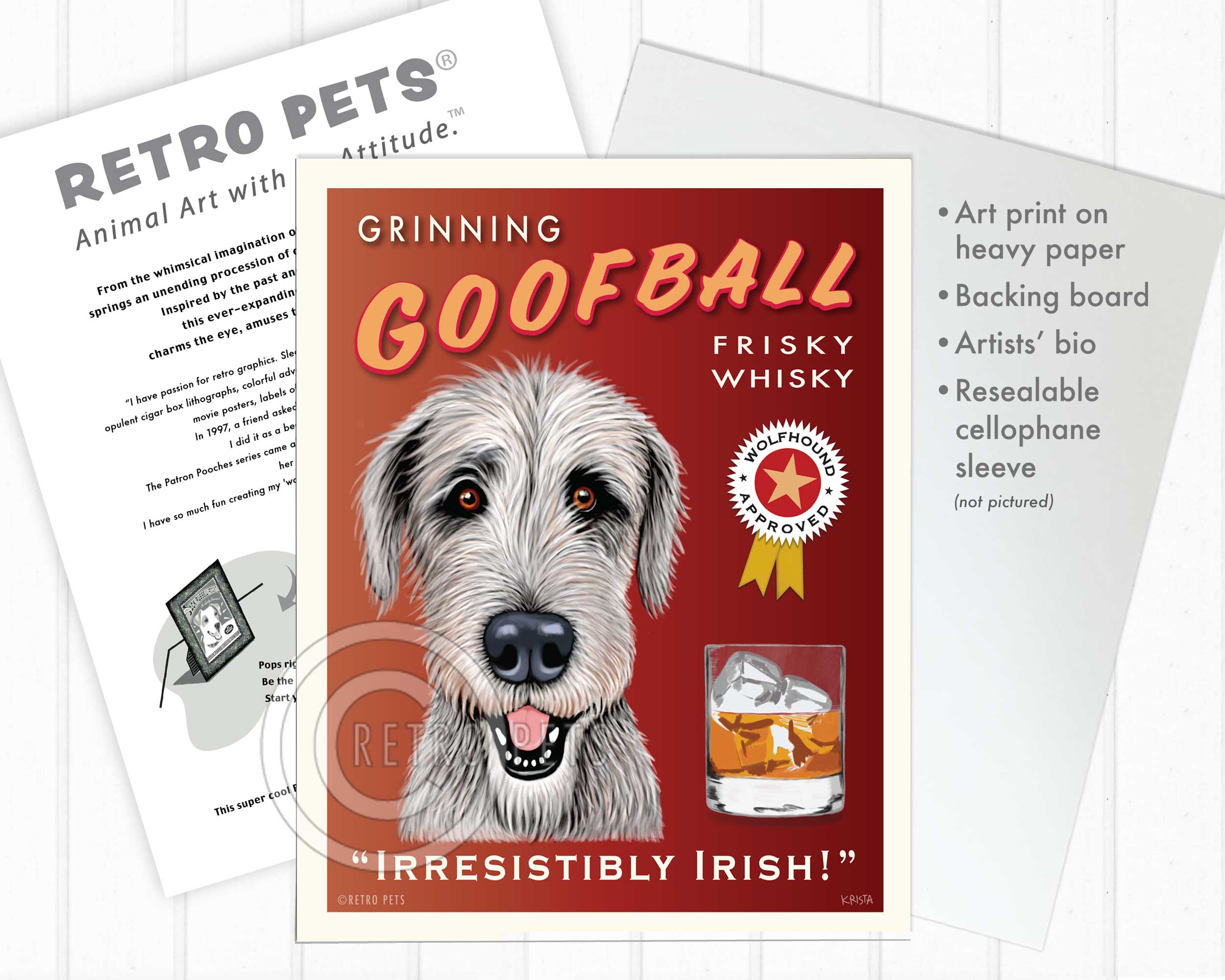The image features a rectangular paper print with a dark red, almost rust-colored background. At its center is a framed portrait of a dog with black and white hair, brown eyes, a black nose, and an open mouth revealing a pink tongue, giving the appearance of a grinning, hairy dog. At the top, in white letters, it says "Grinning," followed by "Goofball" in large orange diagonal letters. Below that, "Frisky Whiskey" is written in bold white all-caps letters. To the right is a starburst design with a white circle, a yellow star in the center, and an orange outer ring, labeled "Wolfhound Approved" with two golden ribbons hanging down. At the bottom of the image, there is a drawing of a whiskey glass with ice and an orange liquid inside. Beneath the glass, the phrase "Irresistibly Irish" is written. The background of the entire scene has a faux paneling texture with light and dark gray tones to simulate a wooden panel. On the left side of this central image, there is additional text indicating "Retro Pets: Animal Art with Attitude," and on the right, a gray piece of paper detailing "Art Print on Heavy Paper Backing Board, Artist's Bio, Resealable Cell Phone Sleeve Not Pictured."